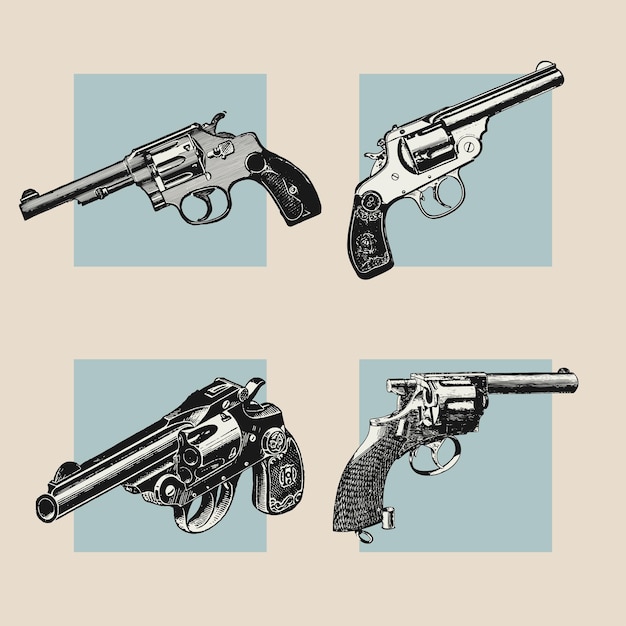The image depicts a digital drawing of four vintage Wild West-style revolvers, each carefully positioned within its own blue square against a pinkish-beige background. The revolvers are rendered in grayscale, exhibiting intricate details. The revolver in the top left corner is angled to the left with a black handle and silver gun portions, while the top right revolver is oriented to the right, featuring a black handle with ornate designs and silver body. The bottom left revolver points diagonally to the left, appearing larger and darker with embellished grips and silver highlights. The bottom right gun, reminiscent of an old cap gun, points to the right with a grayish tone and a distinctively patterned handle. Each revolver embodies the historical essence of firearms from the Wild West era.